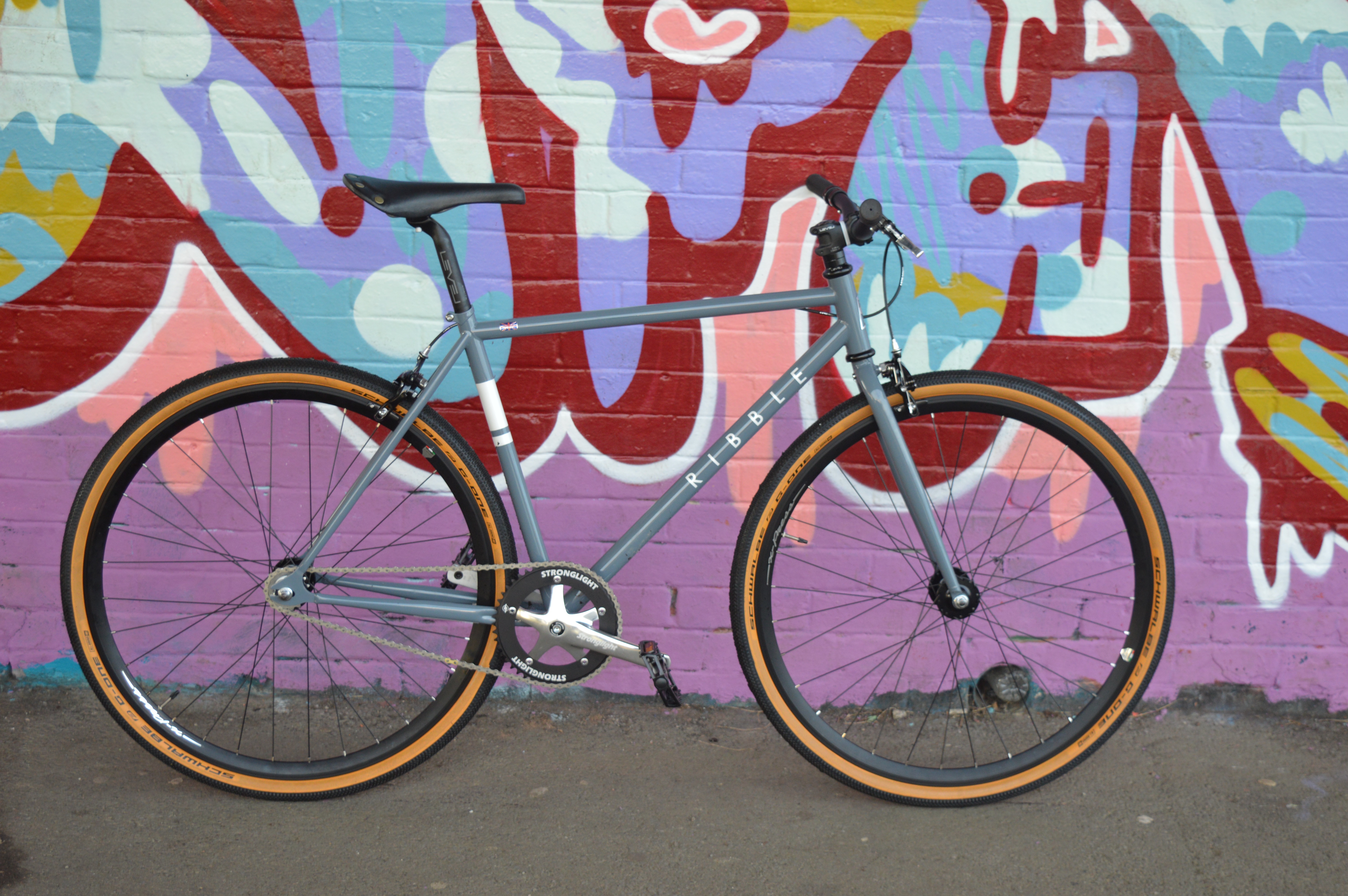The image showcases a Ribble gray bicycle prominently in the foreground, positioned on a grayish-brown concrete pavement. The bike features black tires with distinctive orange sidewalls, a light gray frame, a tall black seat, and black handles. The frame has "Ribble" written in white up the side, and the pedals are branded "Stronglight." Behind the bicycle is a vibrant brick wall adorned with a mural that incorporates abstract shapes and graffiti in a colorful palette, including red 3D elements, along with shades of purple, pink, burgundy, teal, and white. The wall features letters resembling "N" and "Y" in various colors such as white, purple, blue, and yellow, and the base of the wall is predominantly purple. The bicycle is oriented toward the right, standing upright as if ready to be ridden, juxtaposed against the artistic and dynamic backdrop.